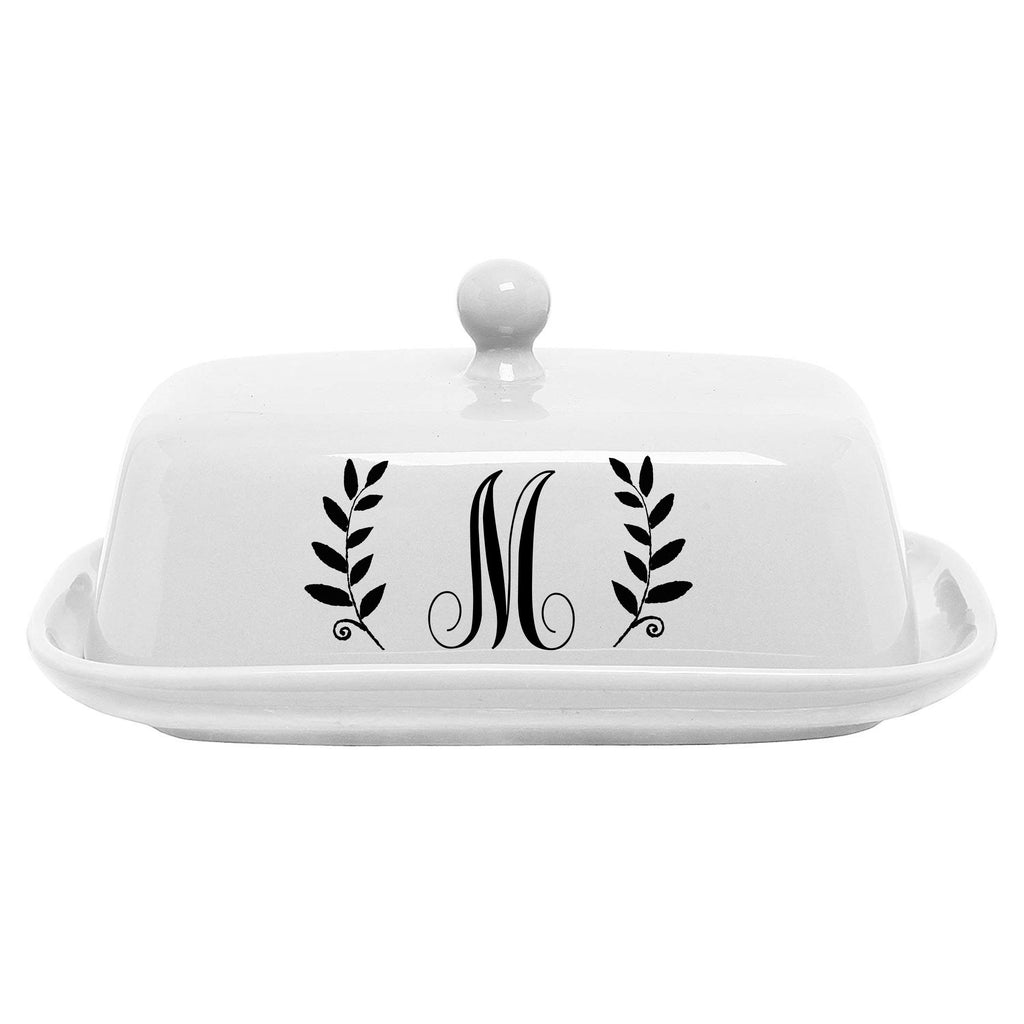The image is a close-up color photograph of a vintage porcelain butter dish, set against a white background. The butter dish is composed of a shiny bright white base and a perfectly fitting rectangular lid with rounded edges. The lid is topped with a small, white, ball-shaped handle for easy removal. The front of the lid features an elegant, black decorative design: a calligraphic capital "M" with pronounced curlicues, flanked on both sides by intricate stems of leaves, each sprig containing multiple rounded, pointed leaves with curlicued ends. The overall dimensions of the dish are approximately six to seven inches in length and two inches in width, giving it a compact yet sophisticated appearance.